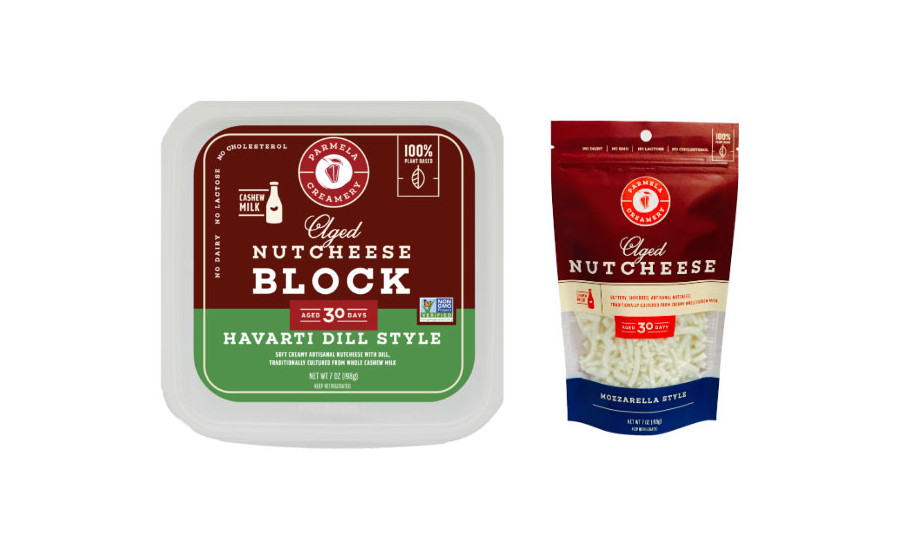Against a pristine white background, the image showcases two products from Parmela Creamery, emphasizing their Aged Nut Cheese varieties. On the left, there is a square plastic container featuring a detailed label. The label's upper half is a dark maroon, while the bottom half is green, stating “Aged Nut Cheese Block” and “Havarti Dill Style” in white text. A prominent red circle logo at the top reads "Parmela Creamery," accompanied by a white bottle icon that mentions "Cashew Milk." 

On the right, a Ziploc bag with a similar dark red upper section and a dark blue bottom houses shredded mozzarella-style nut cheese. The clear middle section of the bag allows a view of the white shredded cheese inside. Both packages prominently display the product name and style, creating a cohesive visual presentation.